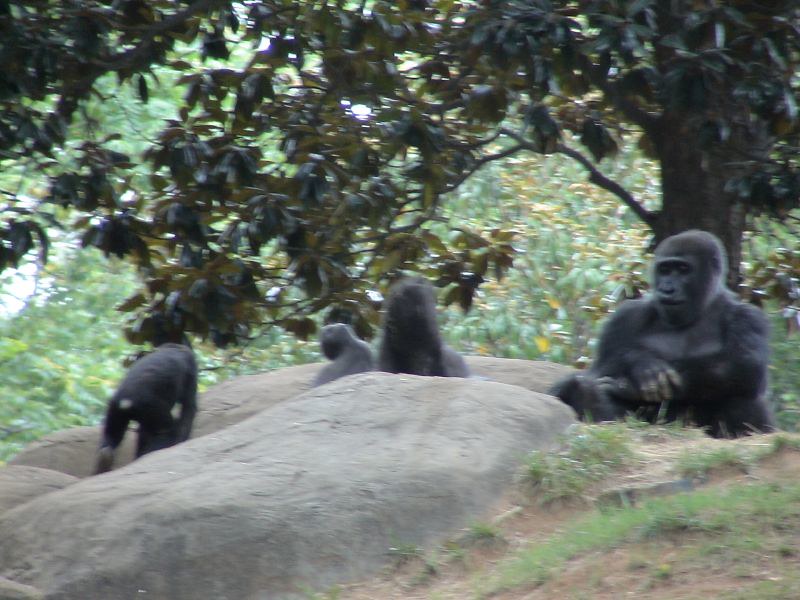This outdoor daytime photograph, slightly out of focus, captures an enclosure with several gorillas amidst a rocky landscape. Central to the right of the image stands a fully grown gorilla, slightly angled in a three-quarter view, looking down with its arms crossed in front of its black, fluffy-furred body. To the left, another smaller gorilla is seen walking away with its back turned, making it difficult to discern finer details due to the blurriness. The image's foreground features a large boulder extending from the left toward the center. On the right side, a sparse grassy hill rises, and a thick-trunked tree with a canopy of green, somewhat floppy leaves provides partial coverage. The lightish sky peeks through the dense leaves, with some yellow leaves intermixed among the green. Behind the foreground gorillas, additional trees of lighter green color fill the distant background, adding depth to the scene.